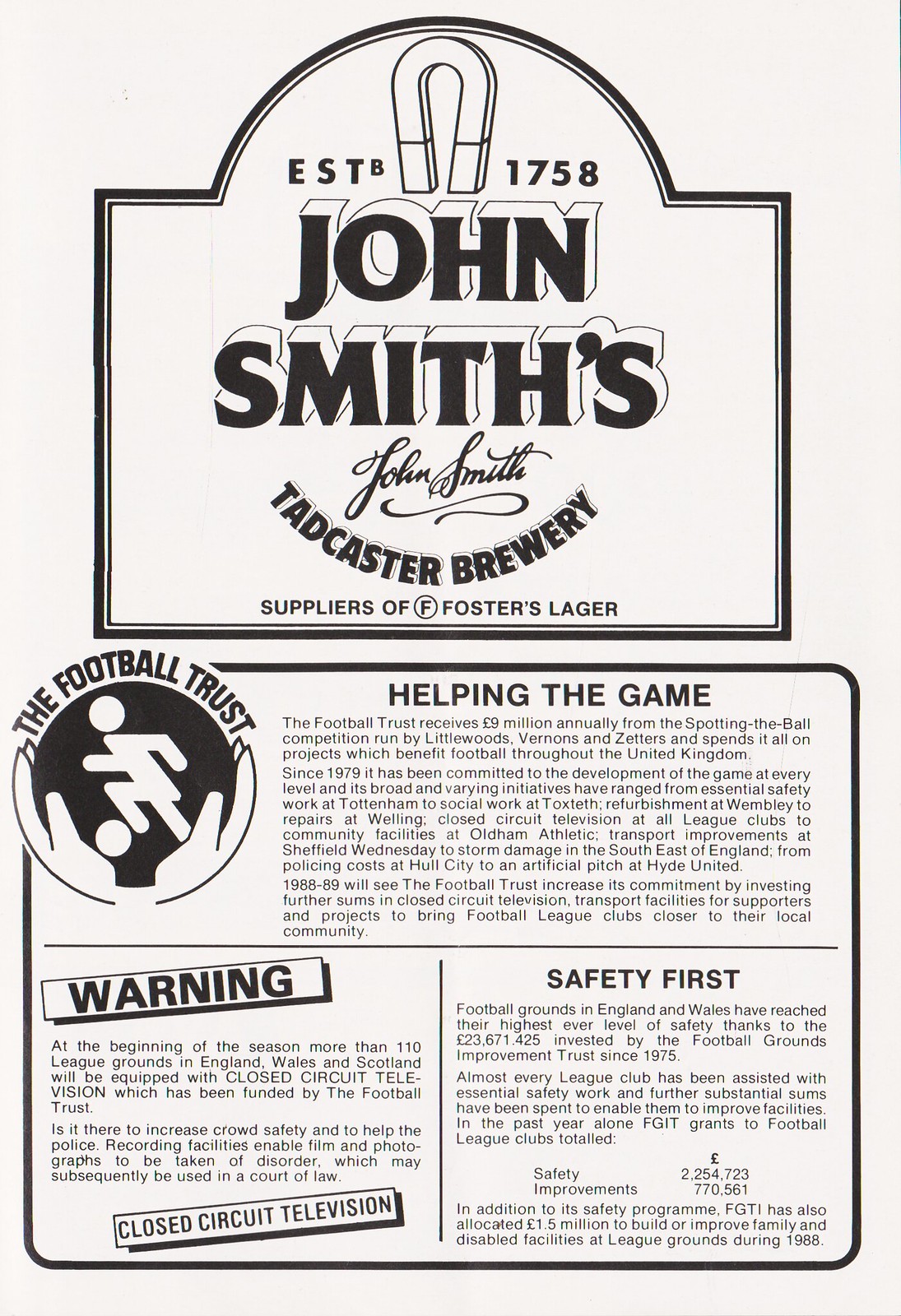This image is a vintage black and white advertisement poster done on white paper, featuring bold black writing. At the top, in a black-bordered header, it reads "ESTB 1758" followed by a large bold "John Smith's" in script font. Below this, it states "Tadcaster Brewery, suppliers of Foster's Lager." Underneath is a prominently bordered rectangle, housing various elements. In the upper corner of this rectangle is a logo depicting two hands holding a soccer player, accompanied by the caption "The Football Trust" and a title that says "Helping the Game." This section includes an explanation of how the Football Trust receives money annually. The lower left corner highlights a warning, mentioning "Closed Circuit Television," while the lower right corner indicates "Safety First." Additional text explains that football grounds in England and Wales have achieved their highest safety levels due to investments from the Football Grounds Improvement Trust since 1975.